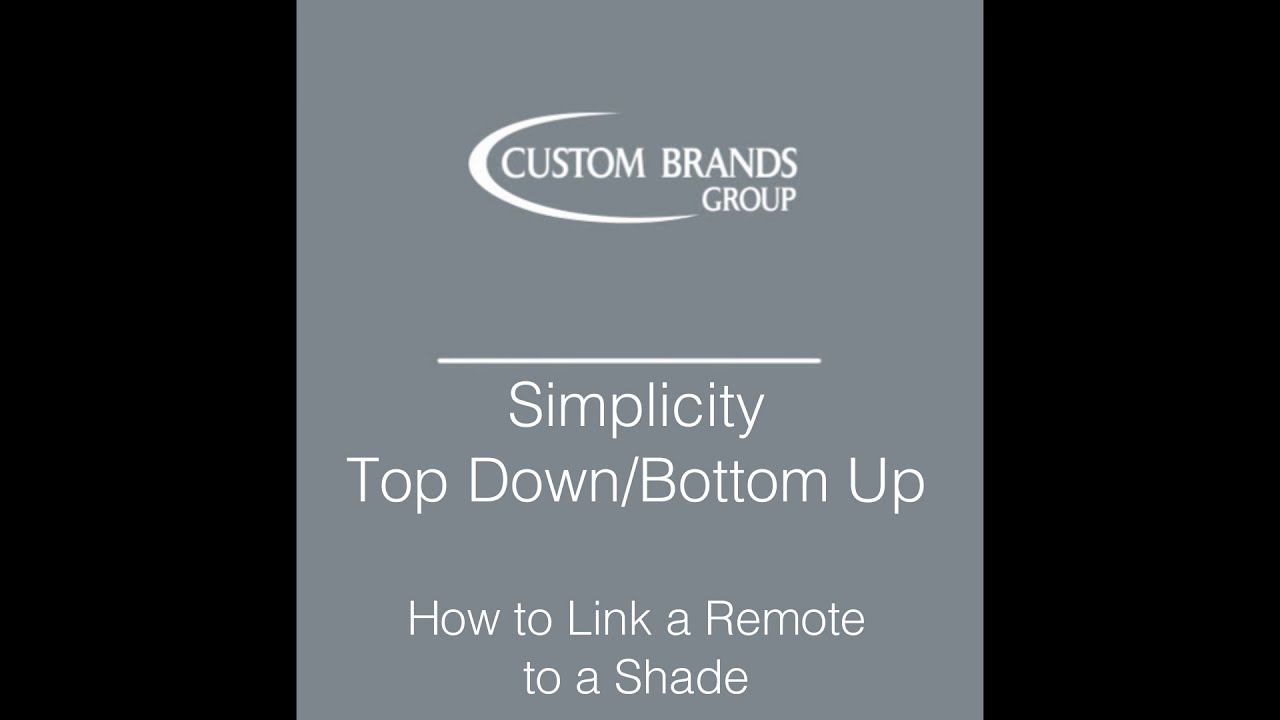The poster features a horizontally rectangular design with thick black trims on both the left and right sides, framing a slightly rectangular, light gray center panel. The top of the gray panel showcases a large, white, crescent-shaped swoosh resembling the letter C, enveloping the white text "Custom Brands Group." Directly below this, a horizontal white line separates the top section from the rest of the content. Beneath the line, the words "Simplicity Top Down / Bottom Up" are prominently displayed in white lettering. Further down, at the bottom of the poster, the white text reads, "How to Link a Remote to a Shade."